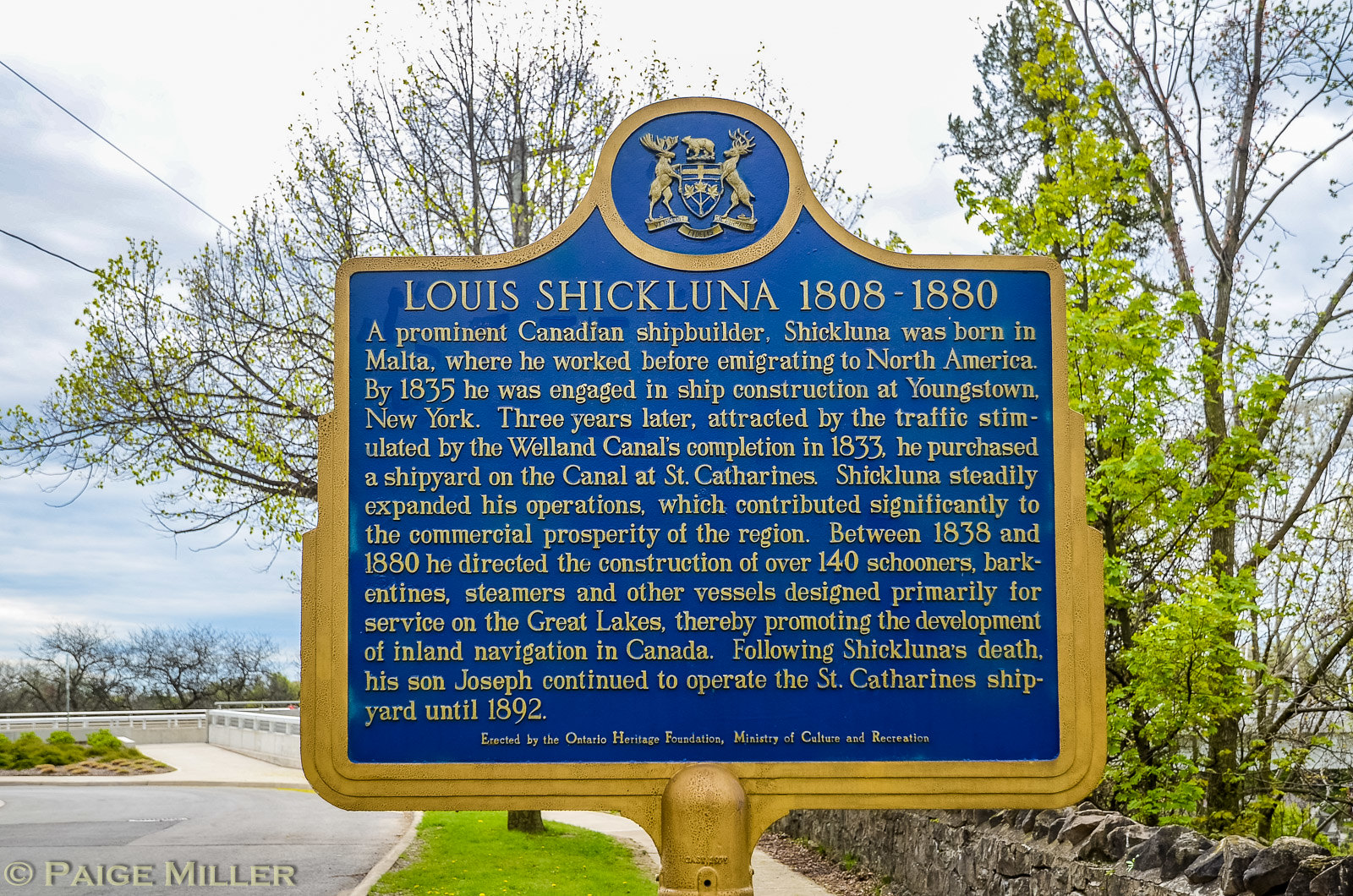The image features a detailed, historical signpost honoring Louis Shickluna (1808-1880), a prominent Canadian shipbuilder. The sign, adorned with a golden emblem and border, has royal blue background and features gold text. Shickluna was born in Malta and emigrated to North America, where, by 1835, he engaged in ship construction in Youngstown, New York. Attracted by the traffic stimulated by the completion of the Welland Canal in 1833, he purchased a shipyard on the canal at St. Catharines three years later. Between 1838 and 1880, he directed the construction of over 140 schooners, barquentines, steamers, and other vessels designed primarily for service on the Great Lakes, significantly contributing to the commercial prosperity of the region and promoting the development of inland navigation in Canada. After Shickluna's death, his son Joseph continued to operate the St. Catharines shipyard until 1892. The sign was erected by the Ontario Heritage Foundation, Ministry of Culture and Recreation. In the background, trees, grass, and a blue sky with clouds can be seen, along with nearby roads and a sidewalk.